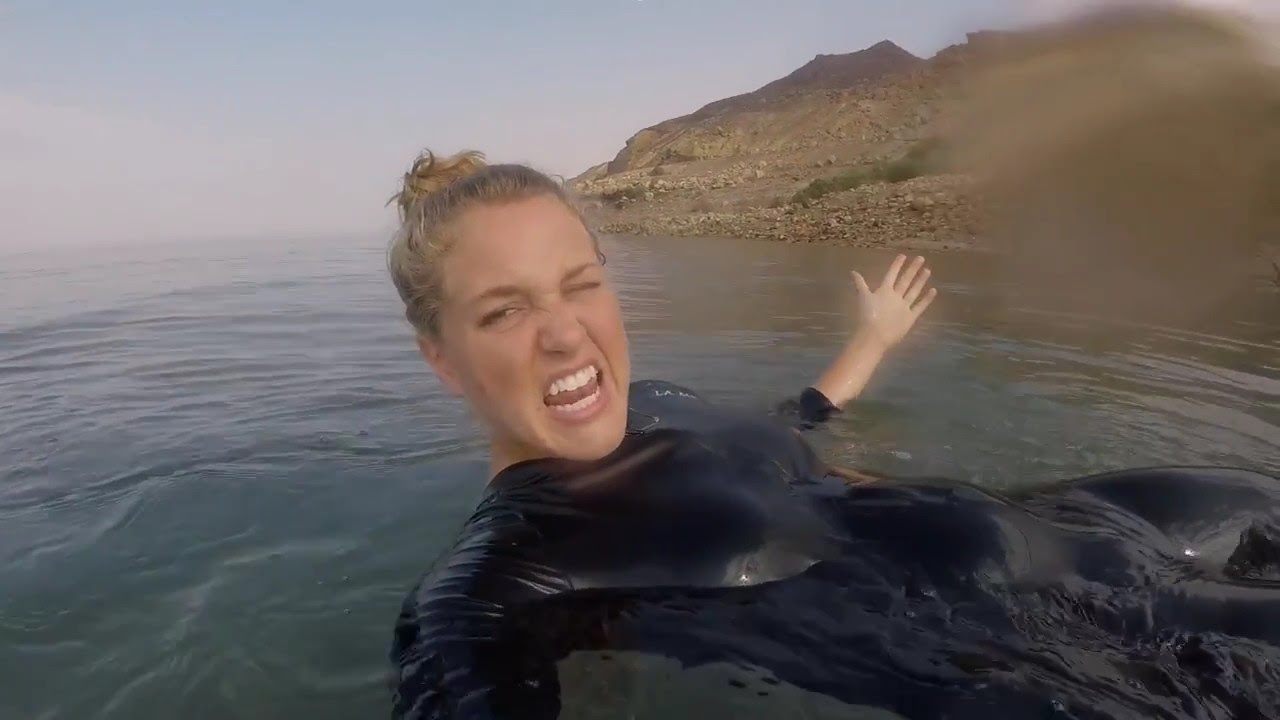In this vivid daytime scene, a blonde Caucasian woman is captured floating on her back in a calm body of gray-blue water, possibly an ocean near a beach. She is wearing a black wetsuit and has her hair tied up in a bun. With one eye closed and her mouth open as if reacting to a splash, she appears to be in motion, swimming backward with her right arm raised. In the background, the horizon stretches under a blue sky dotted with clouds, and a rocky shoreline features a variety of stones in shades of white and light tan, interspersed with small green shrubs and weeds. To the right, a distinctive rocky hill rises, its upper parts displaying a darker, burnt-reddish color. The scene is suffused with natural daylight, though the sun itself is not visible, and there is a hint of fog in the distance, adding to the depth and texture of the environment.